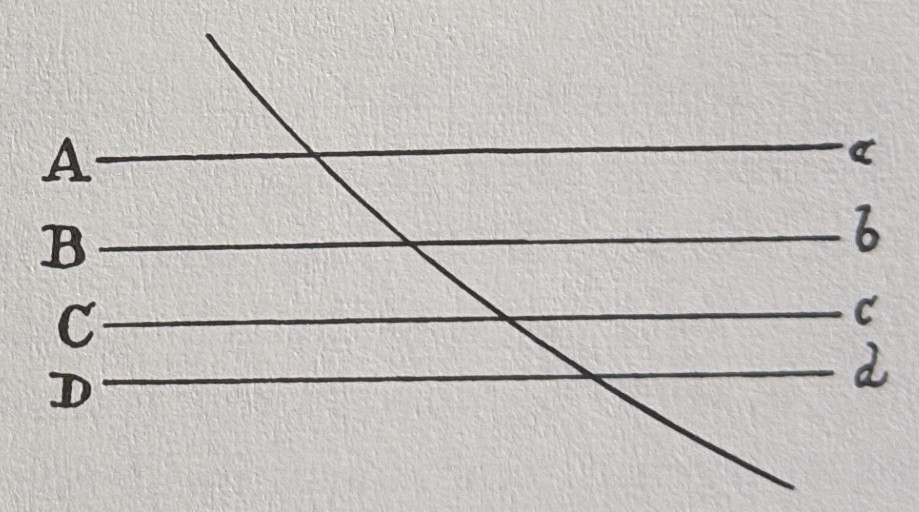This photograph captures an intricately printed image on textured gray cardstock, giving a tactile and vintage aesthetic feel. The composition is structured with four delicate horizontal black lines spanning the width of the image. These lines, evenly spaced, are labeled 'A' through 'D' in uppercase letters on the left side, exuding a straightforward, educational precision reminiscent of a classroom setting.

Intersecting these horizontal lines is a subtle, gently curving line that gracefully arcs from the lower right corner toward the upper left, adding a dynamic element to the otherwise orderly design. This diagonal line brings a sense of movement and complexity, contrasting with the linear regularity.

On the right side of the image, the same four horizontal lines are marked with lowercase letters 'a' through 'd', written in an elegant, old-fashioned script. This script, with its refined, slightly angular stroke, harks back to 19th-century penmanship, bridging the gap between cursive fluidity and block letter rigidity. The juxtaposition of these two styles of lettering, both classic and meticulously crafted, imbues the image with a unique historical charm and visual interest.